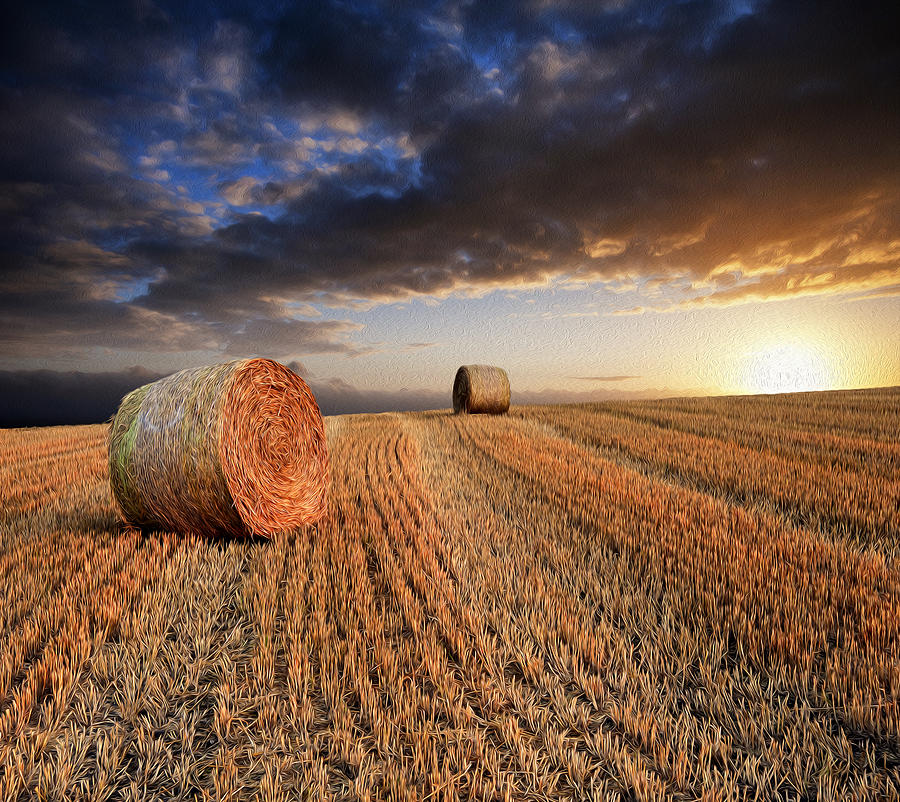This detailed photograph captures a vast, well-kept field of wheat or grain, primarily in shades of brown and light brown, with large circular cylindrical bales of hay scattered across it. Prominent tool marks create defined lines through the rows, accentuating the field's neatness. The expansive field stretches slightly uphill, leading the viewer's eye toward the horizon. At the far end of the field, two hay bales are particularly noticeable—one positioned to the left and another further down towards the center. The time of day appears to be either sunset or sunrise, as suggested by the golden hue bathing the scene. The sky is a dramatic blend of partially cloudy and clear areas. The bottom portion of the sky is clearer, with the sun peeking through, casting its waning light over the landscape. However, dark, almost blackish clouds dominate the upper portion of the sky, creating a stark contrast against patches of vibrant blue. The sun’s rays illuminate parts of the field and the sky, adding depth and warmth to the image.